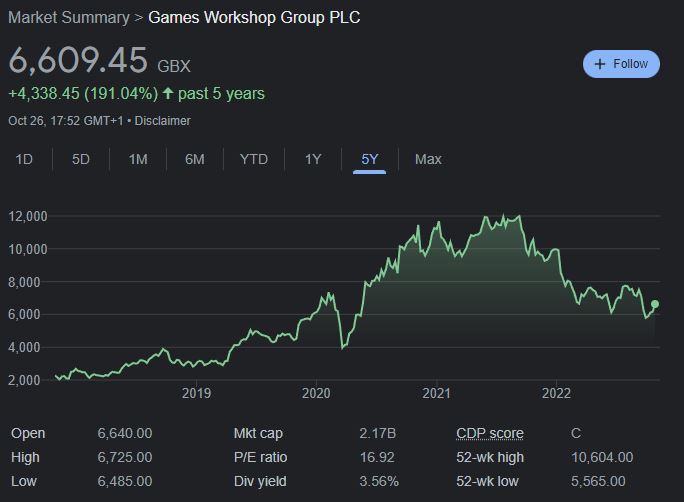This horizontal screenshot captures a stock chart featuring Games Workshop Group PLC, against a jet-black background. The market summary is prominently displayed at the top, with a follow button marked by a plus sign in the upper right-hand corner. The current stock price is indicated as $6,609 or 0.45 GBX. Impressively, the stock has surged by 4,338.45 units of currency, reflecting a remarkable 191.04% increase over the past five years. The chart is set to a five-year view, with vertical markers on the left side displaying values descending from 12,000 to 2,000. Horizontal markers along the bottom denote the years, specifically 2019, 2020, 2021, and 2022, with the chart extending past 2023, although this year is not labeled.

A light green line, shaded underneath to highlight peak values, meanders across the chart, signifying the stock's fluctuating prices over the period. Below this main chart is a detailed listing of various financial metrics: 
- Open, High, and Low prices
- Market Capitalization (Market Cap)
- Price-to-Earnings (P.E.) Ratio
- Dividend Yield
- CDP Score
- 52-Week High at 10,604
- 52-Week Low at 5,565